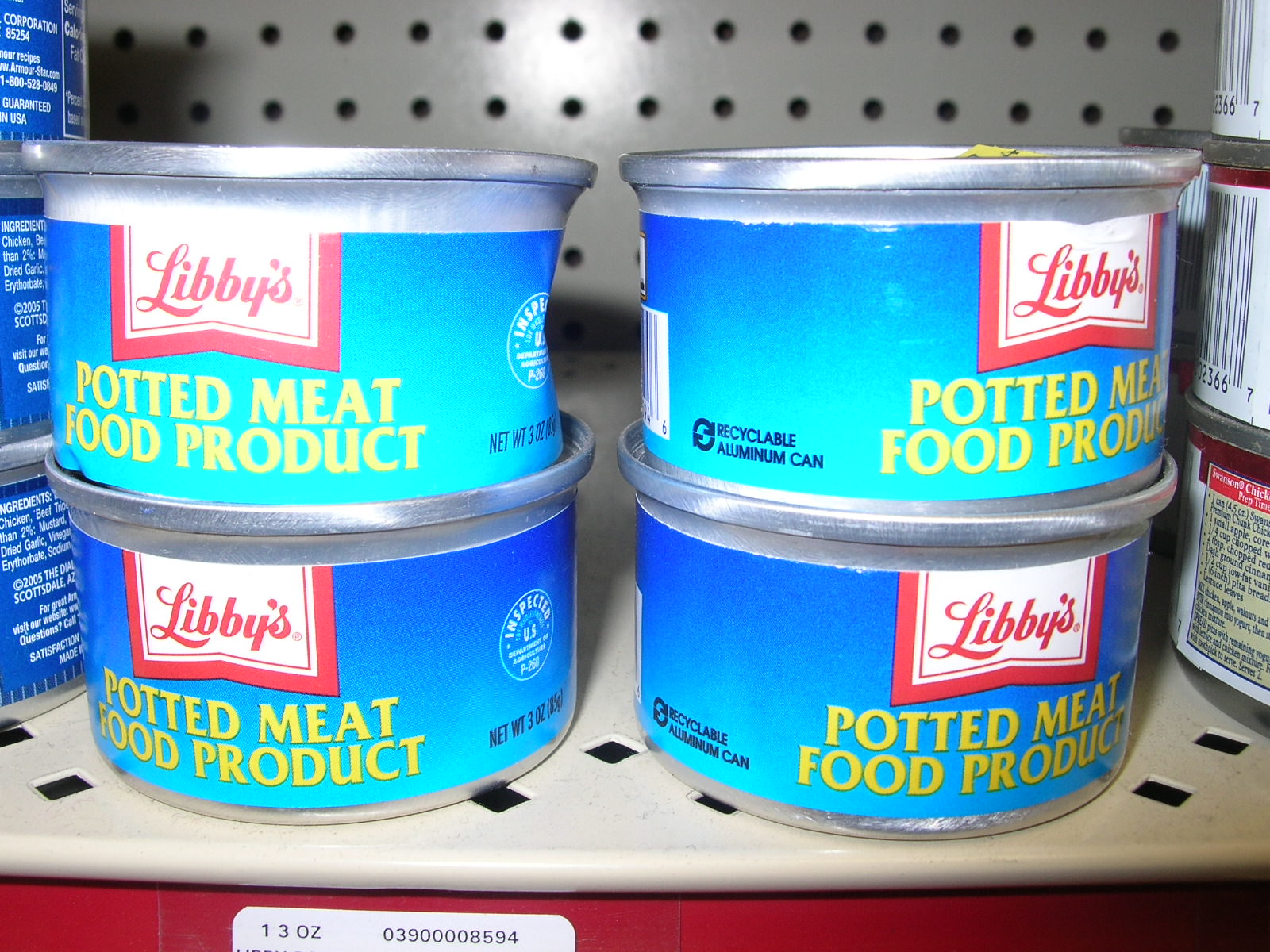This close-up photo captures four identical Libby's potted meat food product cans neatly stacked on a traditional beige grocery store shelf. The cans are arranged in two vertical stacks, each consisting of two cans. The label on each can features a gradient from dark blue at the top to a lighter blue at the bottom. Prominently displayed in the center upper portion of the label is the Libby's logo, with the word 'Libby's' in red over a white background. Directly below the logo, the product name 'POTTED MEAT FOOD PRODUCT' is written in bold yellow capital letters. The cans are made of silver metal and have a pop-off lid similar to tuna cans. The shelf exhibits typical grocery store characteristics with rows of circular and square holes. On either side of the main stacks, partially visible shelves hold additional stacked cans—three predominantly white cans on the left and three blue cans on the right. Below the Libby's cans, the top half of a white barcode that identifies the potted meat is visible, along with a partial sticker indicating it weighs 1.13 ounces.